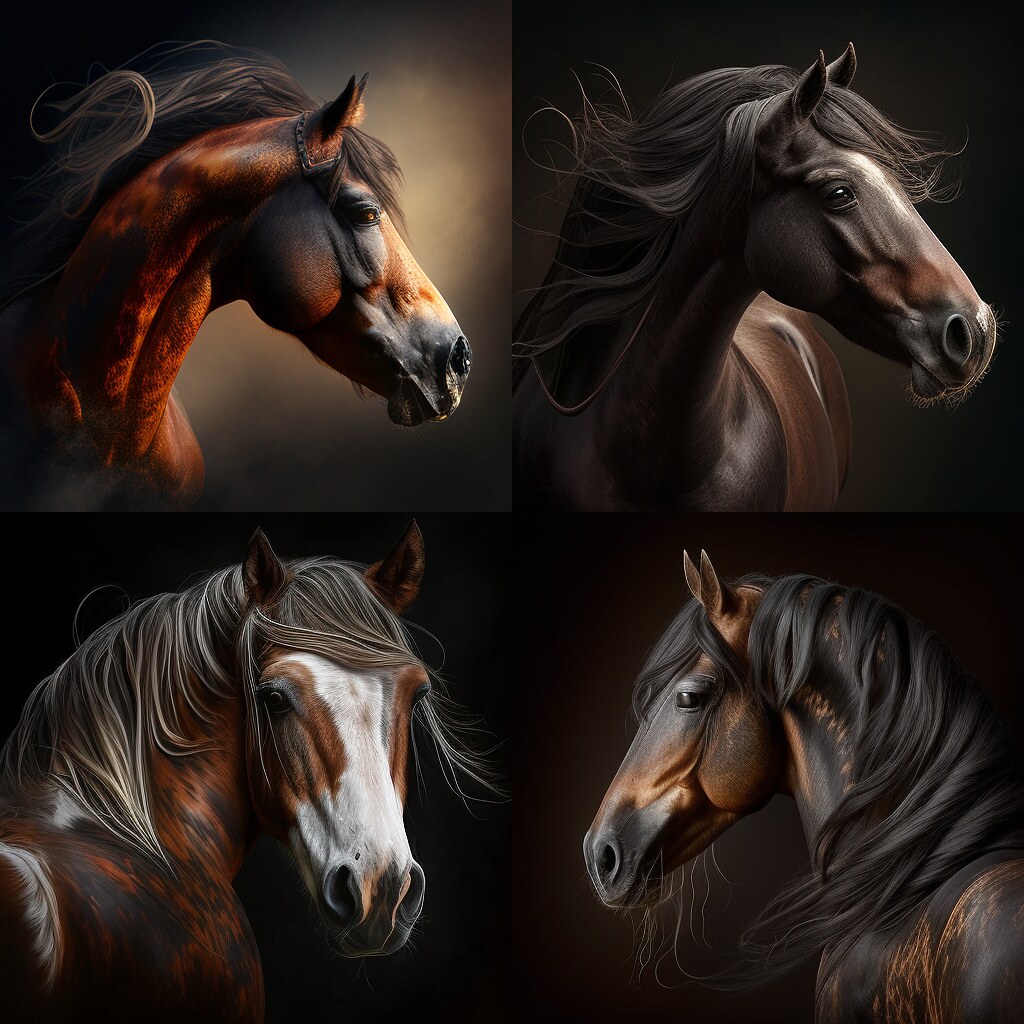The image presents a highly dramatic, AI-generated artwork in a large square format composed of four distinct quadrants, each featuring a lifelike portrait of a horse's head and neck. The backgrounds of all four quadrants are uniform in their dark, almost surreal tones which starkly contrast with the high-detail horse depictions, enhancing the overall dramatic effect. 

In the upper left quadrant, the horse features a burnished orange-brown neck, with dark patterns melding into shades of brown around its eyes and gray around its muzzle, complemented by a dark brown mane. The upper right quadrant portrays a deep burnished chestnut horse, highlighted with lighter shades of brown around its muzzle and neck.

The lower left quadrant displays a horse exhibiting a rich mixture of deep and reddish brown hues. This horse stands out due to a striking white blaze that extends from its forehead down to its muzzle, interwoven with white or gray streaks within its dark mane. Lastly, the lower right showcases a deep brown and golden brown horse with a consistently deep brown mane.

Despite the realistic appearance of the horses, telltale signs of their AI-generated origin can be seen, such as incomplete features—like an interrupted bridle that disconnects and disappears into the image. The overall composition, with its portrait-style dramatic flair, dark backgrounds, and high contrast, lends a surreal, almost otherworldly quality to the artwork, emphasizing the skillful yet unmistakably artificial aspects of its creation.